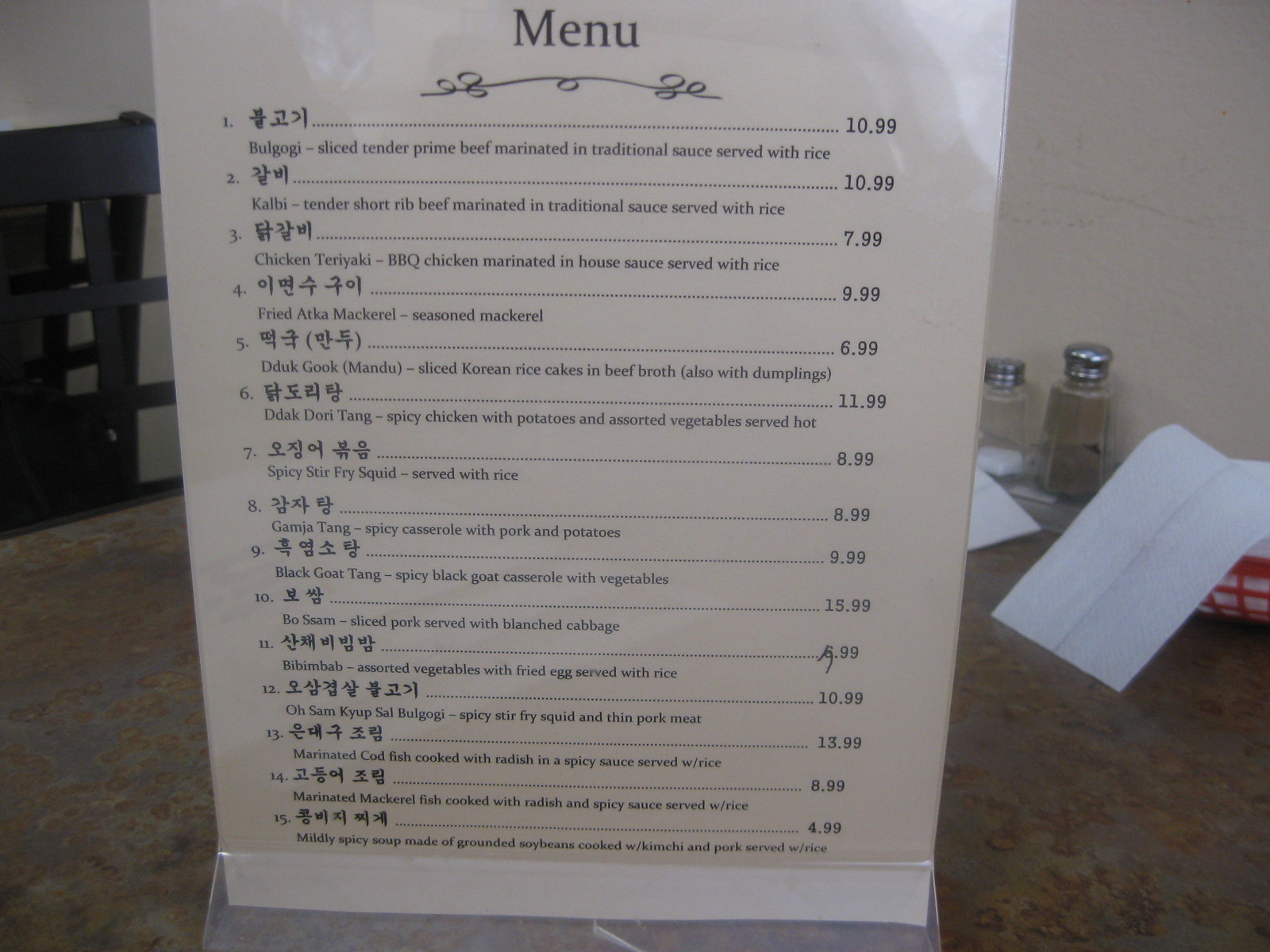The image features a menu encased in a clear acrylic stand, prominently displaying a variety of Korean dishes. The menu is white with black lettering, and the word "Menu" is visibly written at the top above a decorative squiggle.

The first item listed is "Bulgogi," which consists of slivered, tender prime beef marinated in a traditional sauce and served with rice. This dish is priced at $10.99. Below that is "Kalbi," describing marinated short ribs served with rice, also priced at $10.99. The next dish is "Chicken Teriyaki," featuring barbecued chicken marinated in house sauce and accompanied by white rice, priced at $7.99.

Following this, the menu lists "Dduk Gook Mandu," a dish that includes sliced Korean rice cakes in beef broth, priced at $8.99. Another item is "Fried Akitamackerel," a seasoned mackerel priced at $9.99. Also listed is the "Dak-doritang," priced at $8.99. The menu continues with additional items, but the script becomes unreadable towards the end. The final discernible item is priced at $4.99, although the description remains unclear.

In the background, the left side of the image shows the back of a chair, while the right side includes salt and pepper shakers, a napkin, and a red plastic basket lined with paper, typical of restaurant settings.